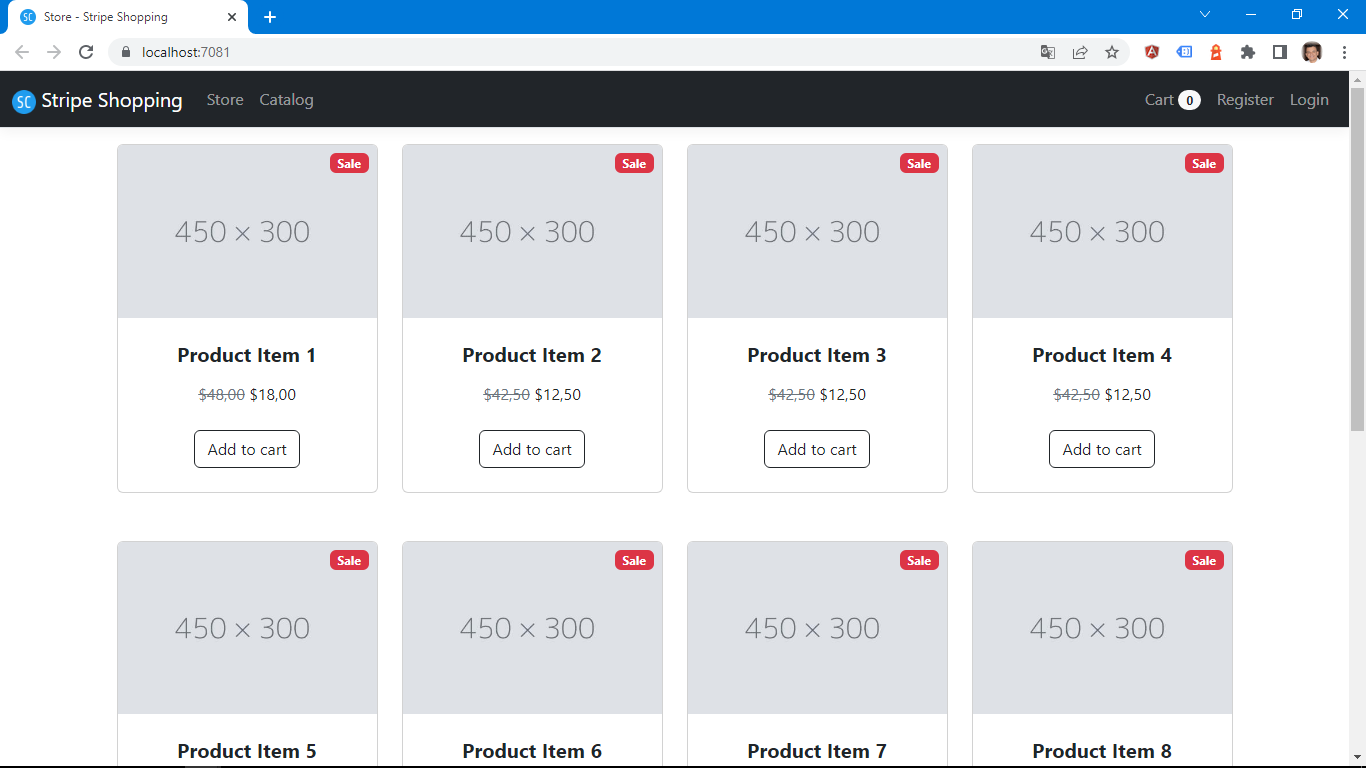This is an image of the Stripe Shopping interface. A black banner stretches from left to right across the top, prominently displaying "Stripe Shopping" in white text alongside a small blue circle featuring an 'S' and a 'C' in white. The banner also includes links labeled "Store Catalog," "Cart," "Register," and "Login." To the right of the "Cart" link, there's a white circle displaying the number 0, indicating an empty cart. 

Above this main banner is a gray search bar labeled "Local Host 7081," and above that, in black text, it reads "Store-Stripe Shopping" next to the same small blue circle with an 'S' and 'C'. Just beneath this, there is another blue banner with a white plus sign on the left and a white 'X' on the right.

Below the main black banner, there is a profile section featuring an individual's profile picture alongside a variety of small icons. The "Store Catalog" displays several product listings. Each product entry includes a placeholder gray box labeled "450 x 300" indicating the image dimensions, and a red "Sale" emblem in the upper right corner.

The first product, "Product Item 1," originally priced at $40, is now listed at $18 with an "Add to cart" button. The second product, "Product Item 2," marked down from $42.50 to $12.50, also features an "Add to cart" button. Similarly, "Product Item 3" and "Product Item 4" are reduced from $42.50 to $12.50.

Further down are more product listings, Items 5 through 8, each within the same "450 x 300" gray placeholders and featuring the red "Sale" emblem. These products are partially cut off by a black line at the bottom, making their details unreadable, but they presumably follow the same pricing pattern and layout as the earlier items.